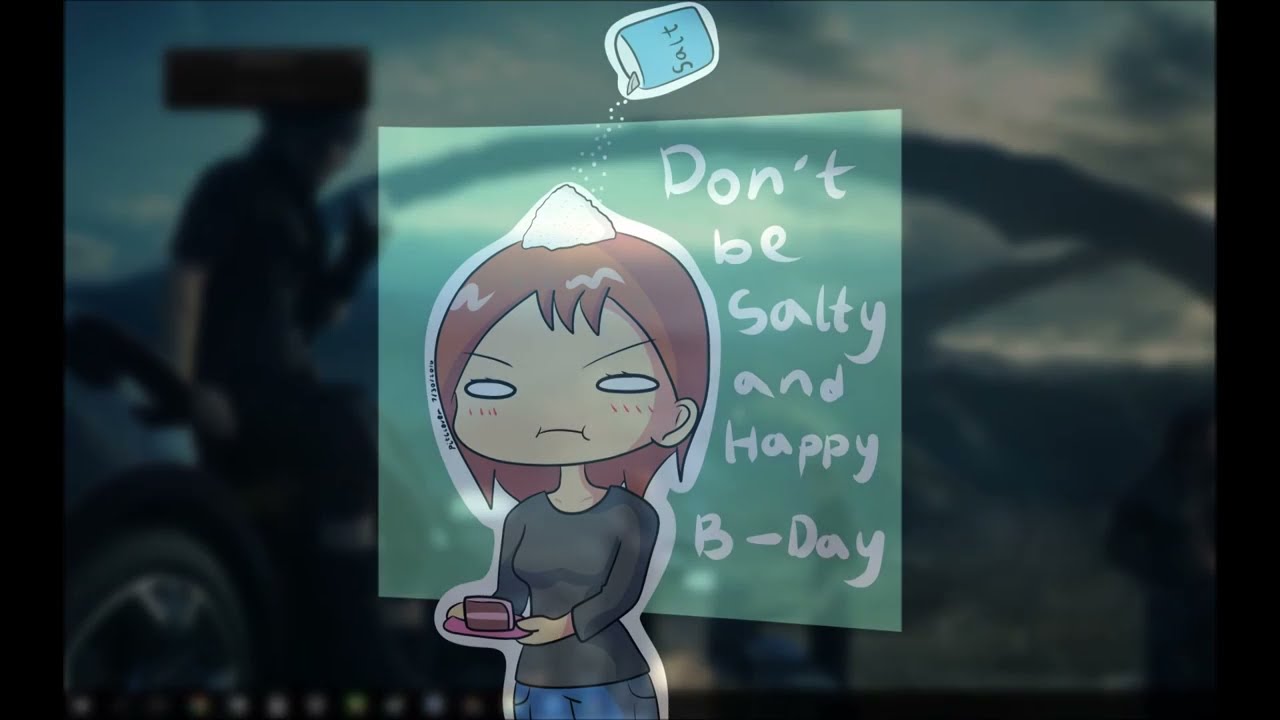In the foreground of the image, there is a humorous birthday card featuring an anime-style drawing of a girl with long brown hair, wearing a gray long-sleeve shirt and blue jeans. She holds a pink plate with a slice of cake decorated with layers of pink frosting and brown cake. Above her, a large salt shaker is sprinkling a considerable amount of salt onto her head, which adds to the comedic effect. The card has the messages "Don't be salty" and "Happy B-day" written beside the girl, who has white, pupil-less eyes and an exaggeratedly large head with a downturned mouth, emphasizing her disgruntled expression.

In the background, partially obscured by the card, is a laptop screen displaying a blurry scene. The screen shows a person standing next to a car, looking out over a mountainous landscape, which can be discerned from the reflection on the laptop's glossy screen. The overall setting appears to be casual, likely at someone's personal workspace. This birthday card, seemingly taped or placed against the laptop, steals the spotlight with its whimsical and highly detailed design.